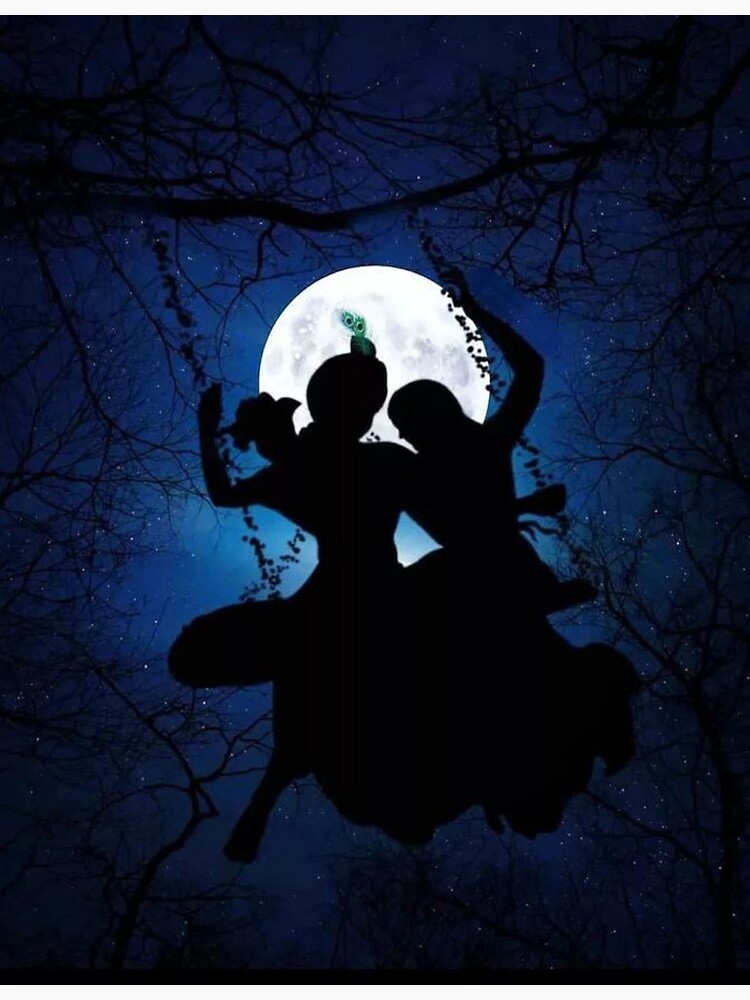In this photograph that appears almost surreal due to its dark and enchanting atmosphere, we observe a young man and a young woman seated on a wooden swing, suspended by ropes adorned with what seem to be flowers, from a large tree branch above them. The scene is dominated by deep blues, giving way to an ethereal ambiance. The focal point of the image is a radiant full moon, casting a bright white glow that silhouettes the couple against the dark night. Both individuals have their backs to the moon, their heads dark against its luminescence. The surrounding sky is speckled with tiny stars, further accentuating the nocturnal setting. The tree branches, stark and devoid of leaves, frame the scene, suggesting a wintry backdrop. One notable detail is a peacock feather-like adornment on the head of the person on the left, adding a touch of color to an otherwise monochromatic depiction.